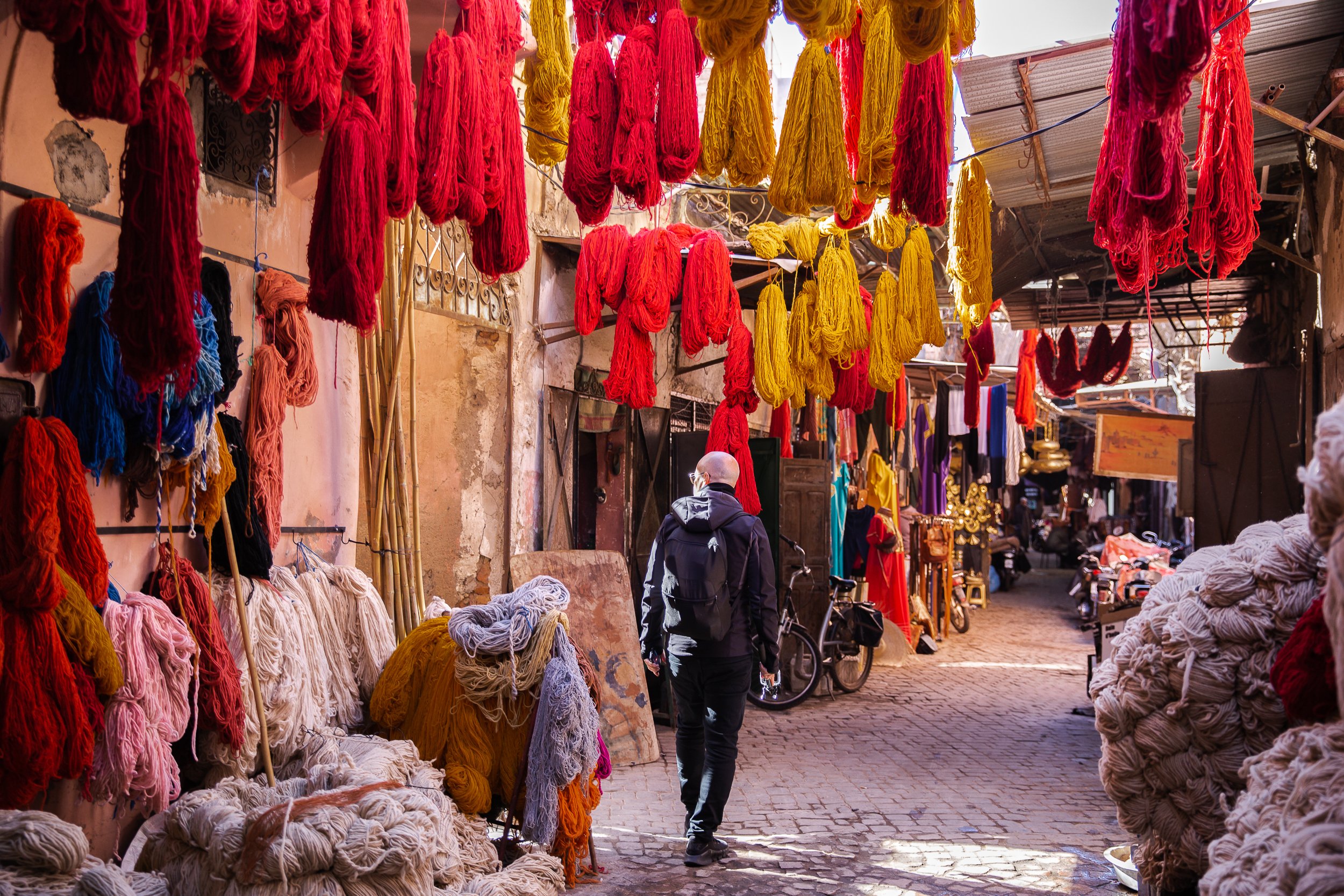The image depicts a bustling street market specializing in textiles, with a narrow, paved path bordered by light white-ish square tiles and cobblestones. Dominating the scene are enormous spools of yarn and ropes in vivid hues of red, yellow, pink, and a variety of other colors, hanging from overhead coverings and strewn on the ground. These yarns and ropes are bundled and organized, suggesting the market is dedicated to textile dyeing or crafting. In the center of the image, a man is walking along the path. He is a mostly bald white man with a smattering of hair stubbles, wearing glasses and dressed in all black, including a black backpack. He's looking towards a brownish door at the back of the market stall path. The market environment is a mix of outdoor and semi-covered areas, with sunlight filtering through the gaps. In the background, additional market stalls and racks of textiles can be seen, contributing to the vibrant and lively atmosphere of this textile-centric marketplace.